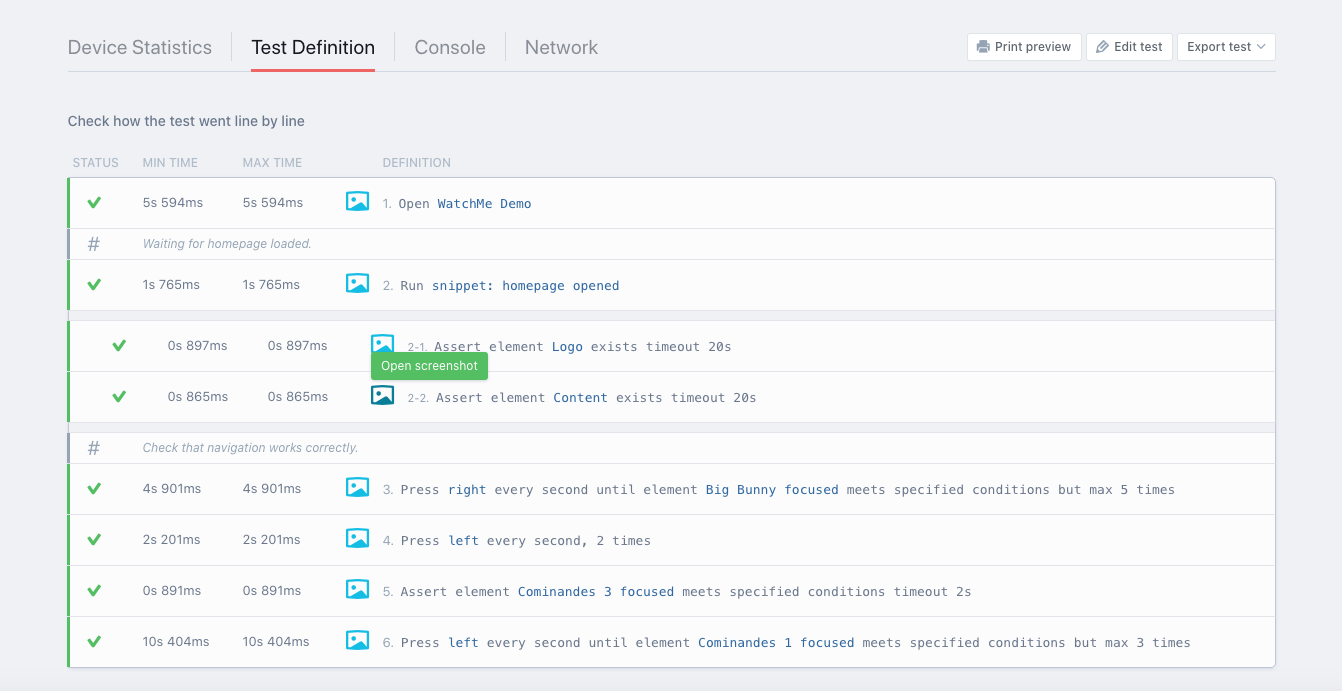The image displays a detailed report from a website testing module. At the top, a navigational panel features buttons labeled "Print Review," "Edit Test," and "Export Test," providing various options for managing the test report. 

The body of the report meticulously documents each step of the website test process. It starts with a record of the user watching a demo and subsequently opening the homepage. For each critical action—namely, "Demo Watched," "Homepage Opened," and subsequent activities—the report includes time intervals that denote the loading duration required for each element, alongside green check marks signifying successful completion.

Additionally, the report is visually supplemented with screenshots corresponding to each milestone, offering a visual timeline of the website's performance and demonstrating the exact state of the website at each recorded interval. This visual and textual combination provides a comprehensive overview for users, likely aimed at facilitating training and quality assurance for website performance.